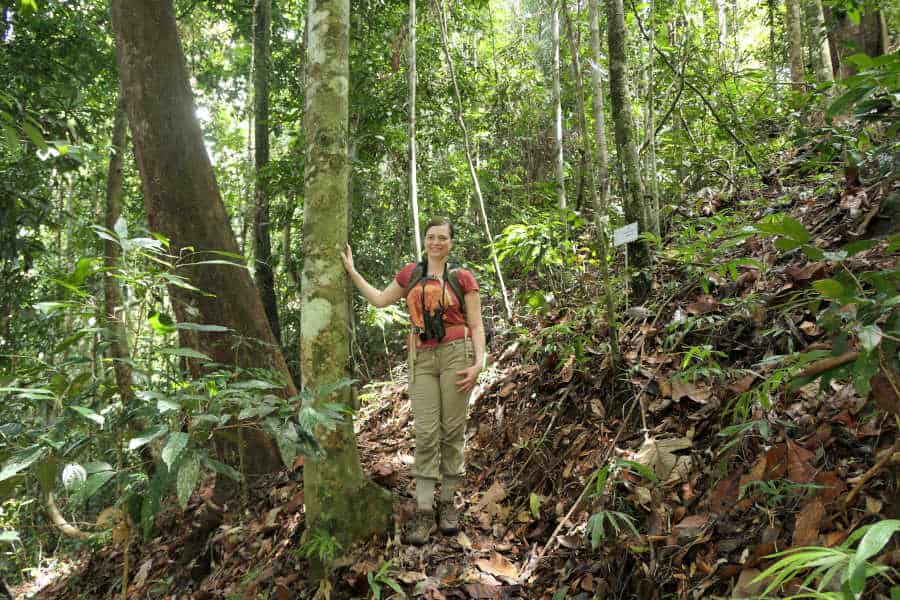In the image, a woman with brown hair tied back is standing in a dense, green forest. She is wearing an orange shirt, tan pants, and brown hiking boots. Around her neck, she has a black camera and possibly binoculars, indicative of her exploring nature. The forest is teeming with trees and greenery, with moss-covered trunks and a ground densely carpeted with dead leaves and brush. The woman leans against a tree, seemingly happy and posing for the photograph. The scene is dominantly earthy with shades of greens and browns, complemented by the woman's vibrant shirt. This photo captures a serene moment of a hiker amidst the tranquil wilderness.